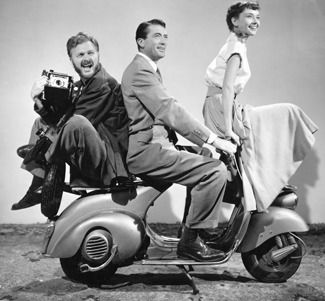This black and white photograph humorously captures a scene with three iconic figures on a vintage Vespa scooter, evoking a nostalgic, old-time movie star charm. The grayscale image features prominent shading towards the bottom, enhancing the monochromatic aesthetic. Audrey Hepburn sits at the front, smiling and looking to her right, attired in a white button-down short-sleeve blouse and a full skirt. Cary Grant, dressed in a light-colored three-piece suit with dark shoes and neatly side-swept hair, navigates the scooter from the middle position, grasping the handlebars. The person on the back of the Vespa, potentially a stand-in for a film set, dons a long jacket, gray pants, and dark shoes. He holds an old-fashioned camera in his hand and has a comically scrunched face with his mouth open and eyes squinted. The entire scene, with its cohesive gray tones and cheerful expressions, appears reminiscent of a classic film, possibly "Roman Holiday."